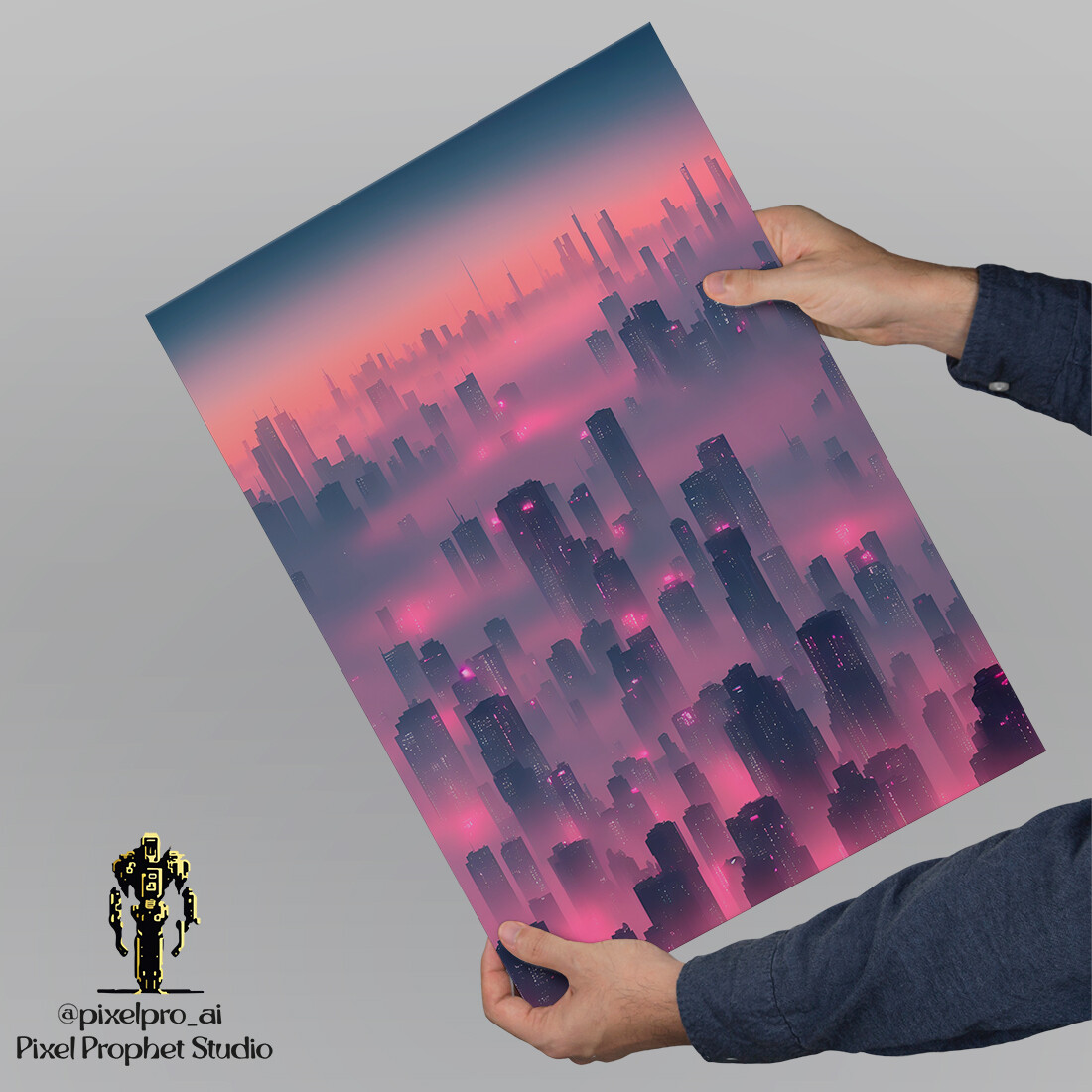A square image features a man with white skin wearing a navy blue long-sleeve button-down shirt, holding a vertical rectangular poster diagonally across the center against a solid medium gray background. The man grasps the bottom-left corner of the poster with one hand and the middle-right side with the other. In the lower left corner of the gray background, there’s a black and yellow robot icon, accompanied by the text "@pixel_pro_AI" and "Pixel Profit Studio" in black print. The poster exhibits a dark blue skyline at the top, transitioning into a gradient of pink and coral hues that form the sky. The foreground showcases a cityscape with numerous skyscrapers, depicted in varying shades of gray and pink, with purple lights adorning their summits. The overall impression of the artwork is a dystopian cityscape, created with a blend of distinct colors and precise architectural outlines.